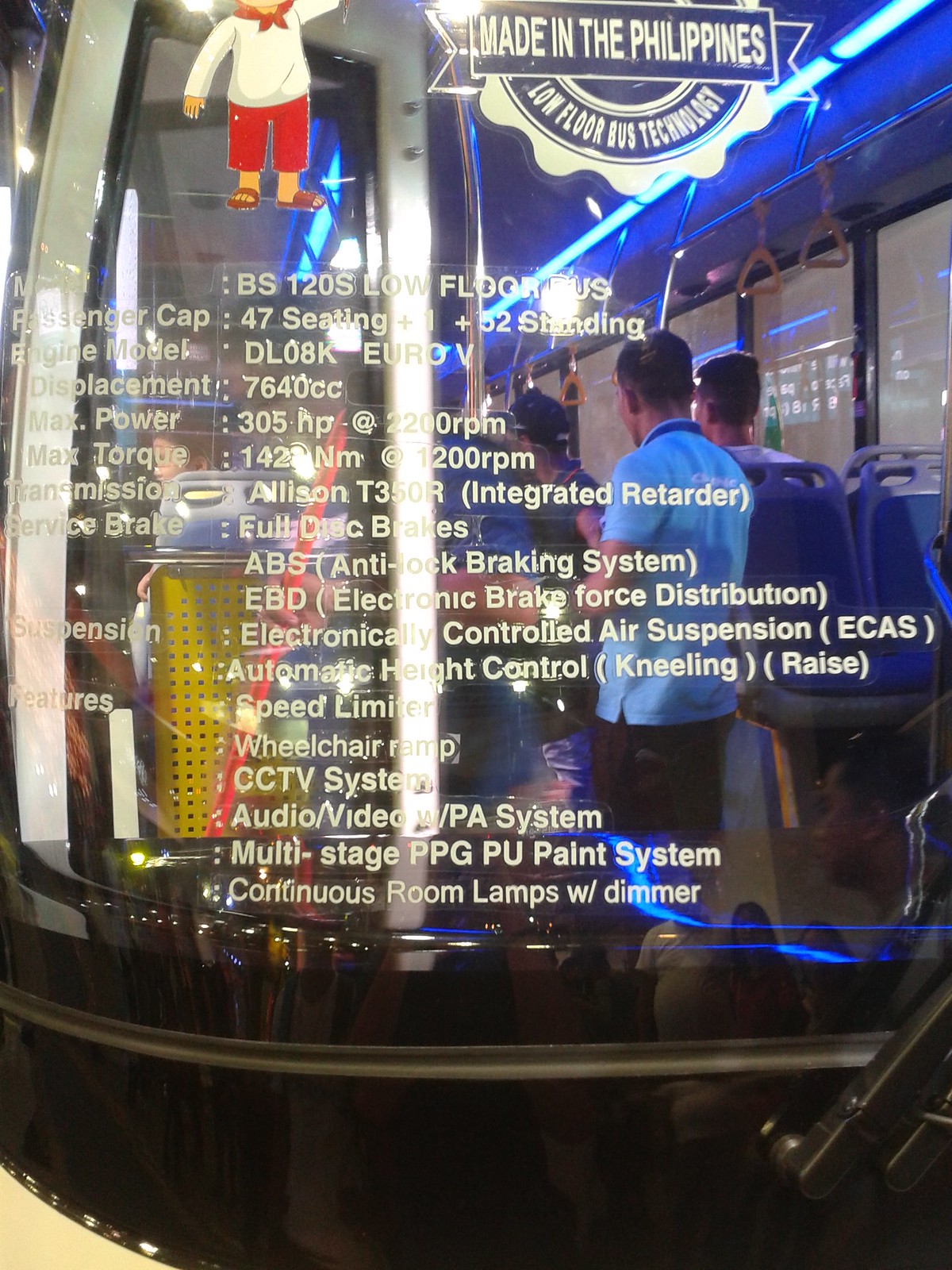This image captures the front portion of a bus, photographed from an exterior angle through its extensive glass front window. The bottom part of the window is black-colored and includes a black windshield wiper visible in the lower right corner, extending upward to the right. Through the transparent window, passengers and blue chairs inside the bus are clearly visible, with blue interior lighting shining through. A man in a blue shirt and black shorts is seen standing inside the bus. The driver's seat is vacant. Prominently displayed at the top center of the window is a blue banner with white text that reads "Made in the Philippines Lo-Floor Bus Technology." Additionally, there is a cartoon-like drawing of a man dressed in red pants, a white long shirt, and red sandals, situated at the top right. The window is covered with detailed white text specifying the bus's characteristics, including the model "BS120S Lo-Floor Bus," passenger capacity of "47 seating plus 1 plus 52 standing," engine model "DL08K Euro V" with displacement "7640 cc," and maximum power "305 HP at 2200 rpm." Other features include the "Allison T350R Integrated Retarder," "ABS Anti-lock Braking System," "EBD Electronic Brake Force Distribution," "electronically controlled air suspension (ECAS)," "automatic height control kneeling arrays," "speed limiter," "wheelchair ramp," "CCTV system," "audio-video PA system," "multi-stage PPG PU paint system," and "continuous room lamps with dimmer." This comprehensive assortment of detailed specifications describes the bus's advanced technological features and performance capabilities.